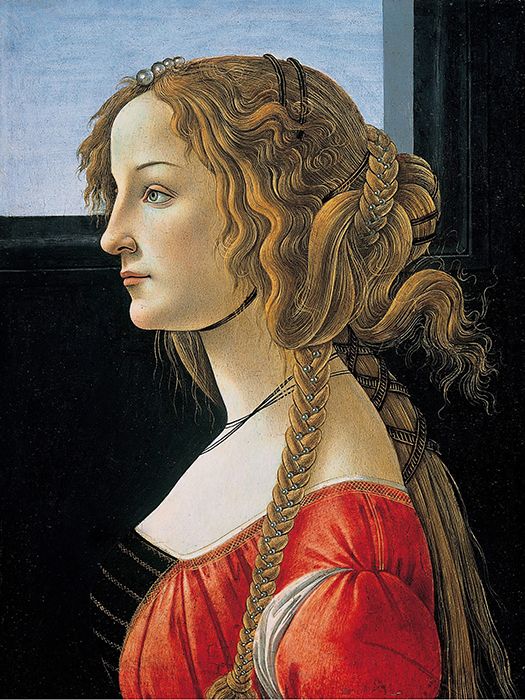This detailed illustration depicts a woman from the 1800s, possibly of European descent, with fair to peach-colored skin and striking blue eyes. Her sophisticated hairstyle includes reddish auburn, almost strawberry blonde hair, which is partially braided and adorned with jewels. The top part of her hair forms a half bun wrapped with a braid, while the rest cascades down freely, secured by a ribbon, with some strands curling slightly. Additionally, a long braid embellished with small jewels descends from the front. She wears an elaborate red dress featuring a black velvet section near the bust, complemented by a necklace. The background comprises a dark, almost black wall and a window revealing a clear blue sky. The woman's profile is turned to the left, showcasing her Roman nose and an expression poised between a smile and a frown, indicative of serene composure. This composition evokes a Renaissance aesthetic, emphasizing the woman's elegant attire and poised presence.